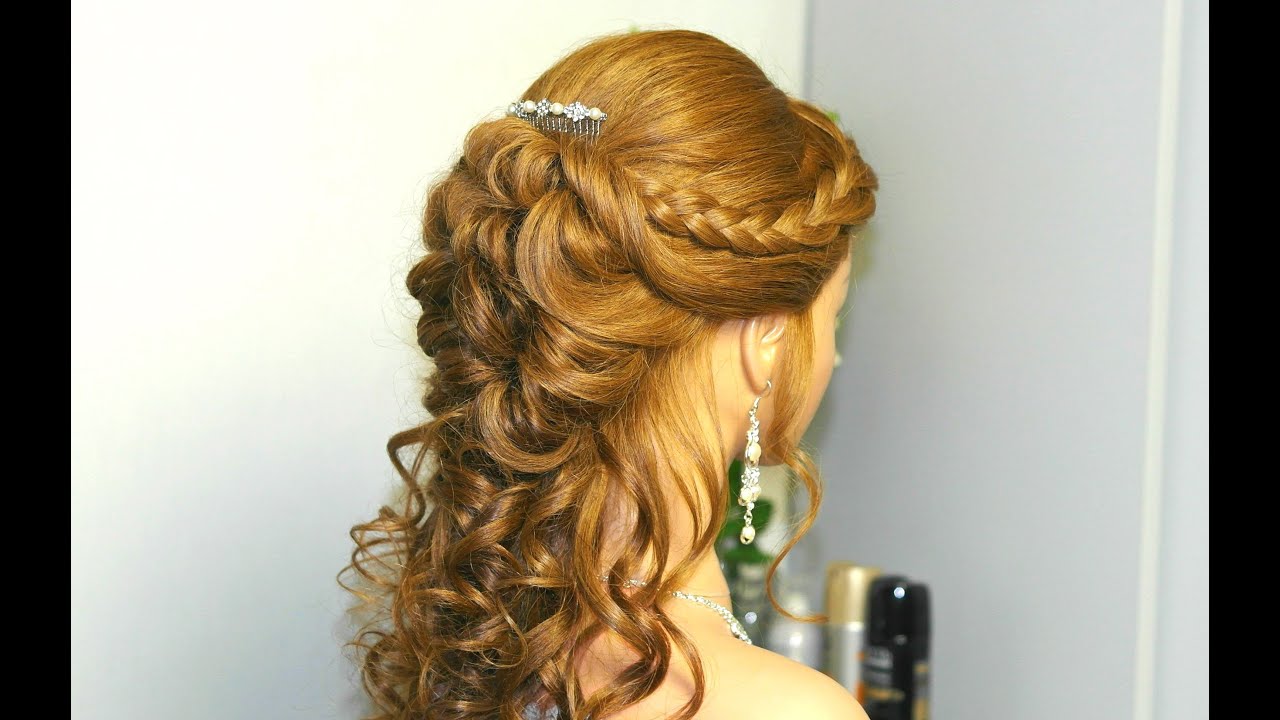In the photograph, a woman with stunning red hair is shown from the back, possibly preparing for a special occasion like a wedding or prom. Her richly colored hair cascades in soft curls down her back and shoulders, interwoven with braids that crown her head. These braids are held in place by a sparkling comb adorned with diamonds and pearls. On her right ear, she wears an elegant, long, dangling earring featuring crystals and pearls, which matches her exquisite crystal necklace. Her fair skin is illuminated in the image, enhancing the look of sophistication and grace. The backdrop reveals a plain room, blurred but hinting at beauty products like hairspray cans, suggesting she might be standing in a bathroom. Overall, it is a meticulously crafted hairstyle captured in a serene moment before the special event.